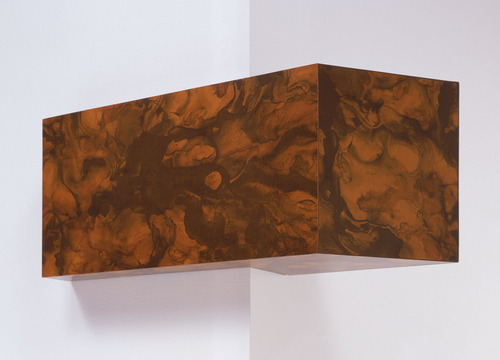The image showcases a computer-generated scene featuring two intersecting white walls, one slightly off-white, creating a central demarcation line where they meet near the middle of the frame. Affixed at the corner of this intersection is a rectangular wooden block with a rich mahogany, burl-like appearance, adorned with darker and lighter brown abstract patterns. The rectangular block’s square face is oriented towards the right side of the image, and its complex marbled finish might suggest a decorative or design object, potentially part of an advertisement for furniture or interior design, highlighting the texture and color options available. The overall look is clean, modern, and slightly ambiguous, hinting at a suspended or uniquely mounted placement of the block, adding an element of visual intrigue.